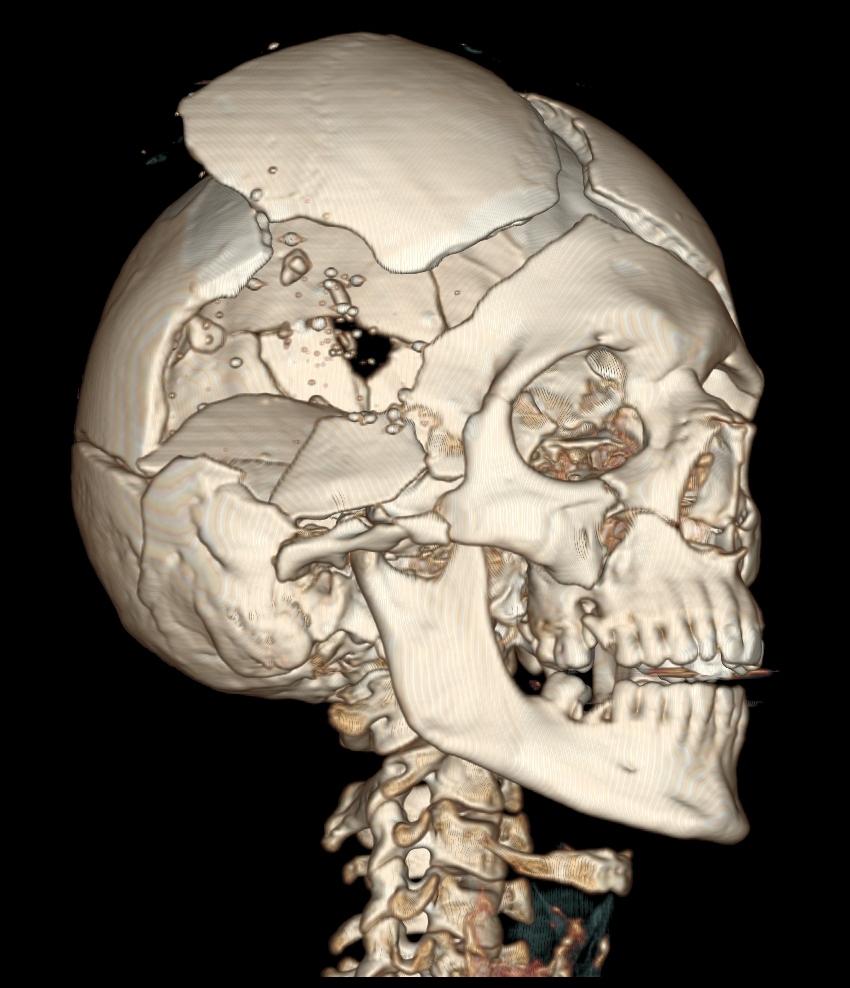This detailed artwork features a surreal, computer-generated image of a human skull and the upper section of a spinal column, set against an all-black background. The skull, rendered predominantly in white with reddish, beige, and brown hues, exhibits an intriguing blend of anatomical realism and abstract artistic elements. The cranium is fractured, with pieces at the top and the right side appearing to break apart and float away, resembling puzzle pieces or liquid fragments. The eye sockets reveal complex inner details rather than voids, contributing to the sense of a partially deconstructed anatomy. Connecting to the neck, the spinal column is visible, reinforcing the anatomical theme. This striking piece melds precise detail with imaginative deconstruction, evoking a sense of both decay and intricate structure.